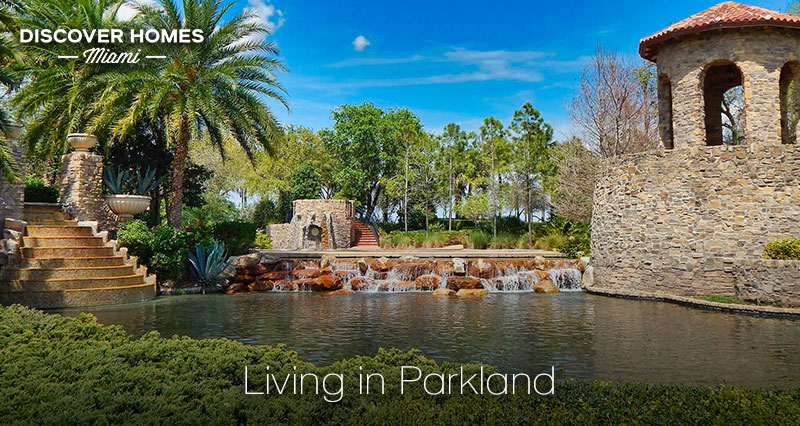This photograph, likely a magazine insert meant to span two pages, showcases a picturesque scene from Discover Homes Miami with the caption "Living in Parkland" at the bottom in white typeset. The image features a large, serene body of water, possibly a decorative pool or pond, framed by lush greenery and ornate structures. To the top left corner, the title "Discover Homes" is prominently displayed in black and white typeset with the word "Miami" in italics below.

On the left side of the photograph, elegant stairs descend towards the water's edge, flanked by majestic palm trees and verdant bushes. A stunning waterfall cascades over river rocks at the center, creating a captivating focal point. Adjacent to this, another smaller set of stairs ascends next to a striking stone building.

To the right, a brown stone gazebo with a Spanish tile roof and cylindrical shape is situated, almost as if encircling the water like a moat. This structure, likely a public feature, adds a touch of grandeur to the scene. The photograph captures the tranquil atmosphere of late afternoon, with the sun casting gentle shadows and reflections on the water. In the background, various trees, including more palm trees, complete the idyllic landscape.